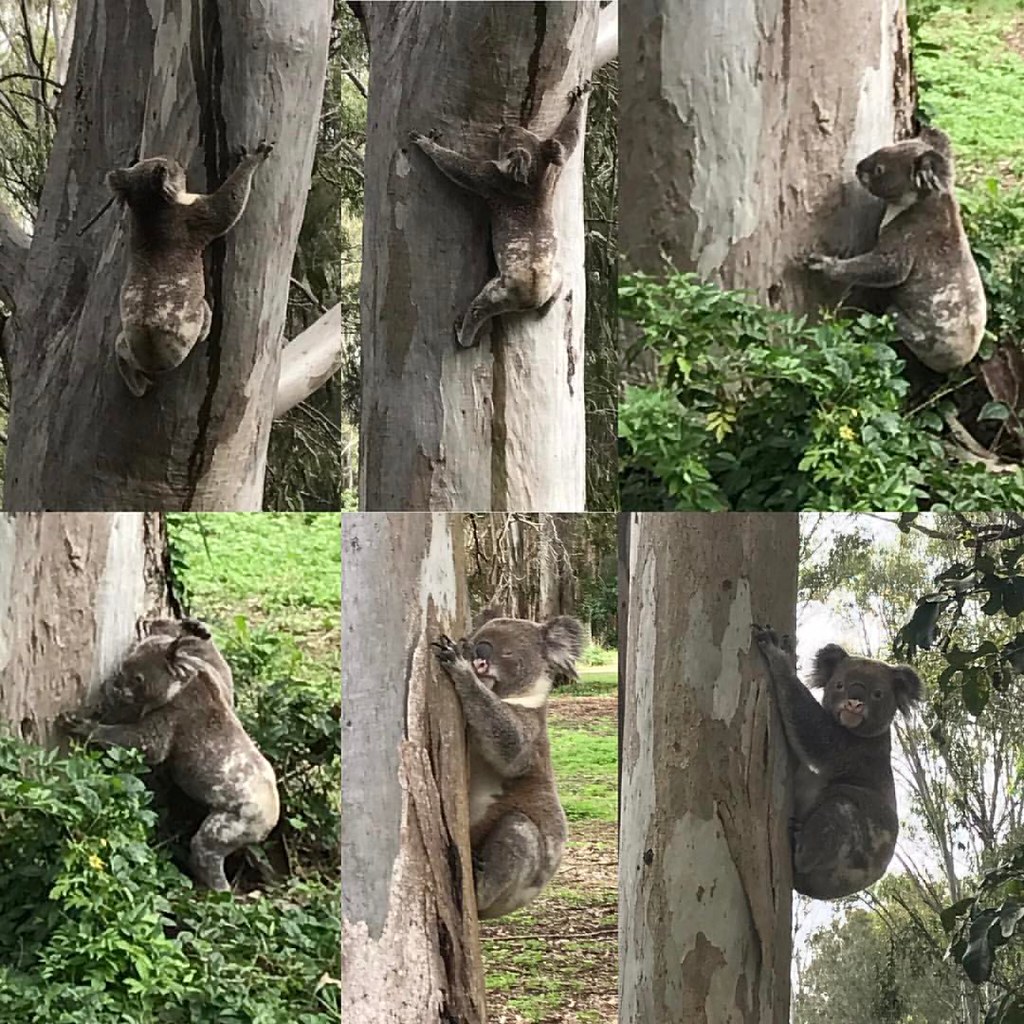In the image, we see a sequence of two vertically stacked pictures showcasing six koalas amidst a grassy setting with multiple trees. Each koala is engaged in various actions on the grayish-barked trees. 

In the top row, there are three koalas interacting with the trees: 
1. The koala on the far left is viewed from behind, clinging to the tree trunk with its claws dug in.
2. The middle koala is also clinging to the tree, with its eyes closed and facing towards the tree.
3. The far-right koala is looking forward with its claws dug into the tree, seemingly holding on tightly.

In the bottom row, the scene continues with three more koalas:
1. The koala on the far left is near the base of the tree, beginning to climb upward.
2. The middle koala is climbing up and looking skyward, with its limbs outstretched in an ascending motion.
3. The far-right koala, higher up the tree and facing the camera, shows a clear view of its face and eyes, appearing content and immersed in its climb.

Together, these images form a detailed and engaging montage capturing the diverse postures and activities of koalas on the trees, surrounded by a lush backdrop of grass and green leaves.